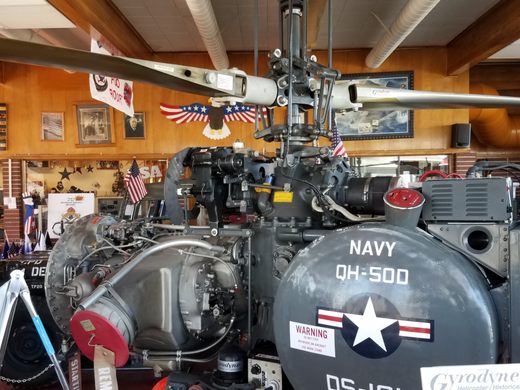The image depicts an indoor scene within what appears to be an aircraft or military museum, potentially doubling as a workshop. The room has wooden paneling on the back wall, adorned with numerous framed photographs and a decorative eagle with red, white, and blue wings, embodying a patriotic theme. Supporting the ceiling are heavy wooden beams and round plastic ducts, along with tube lights illuminating the space.

Prominently featured in the foreground is a complex, gray metal object, identified as part of a military helicopter engine or a model helicopter. This object bears intricate extrusions and operational components, including a large round, shallow extrusion resembling a garbage can lid. This feature is adorned with a Navy Air Forces logo and the designation "Navy QH-500". The helicopter component showcases a mix of gray painted and silver metal parts, interconnected by a network of silver tubing. Above this setup, a shaft extends to white propeller blades, denoting the helicopter's rotor system.

Overall, the scene is one of organized clutter, reflecting a blend of historical reverence and mechanical fascination, marked by the presence of various American flags and memorabilia.